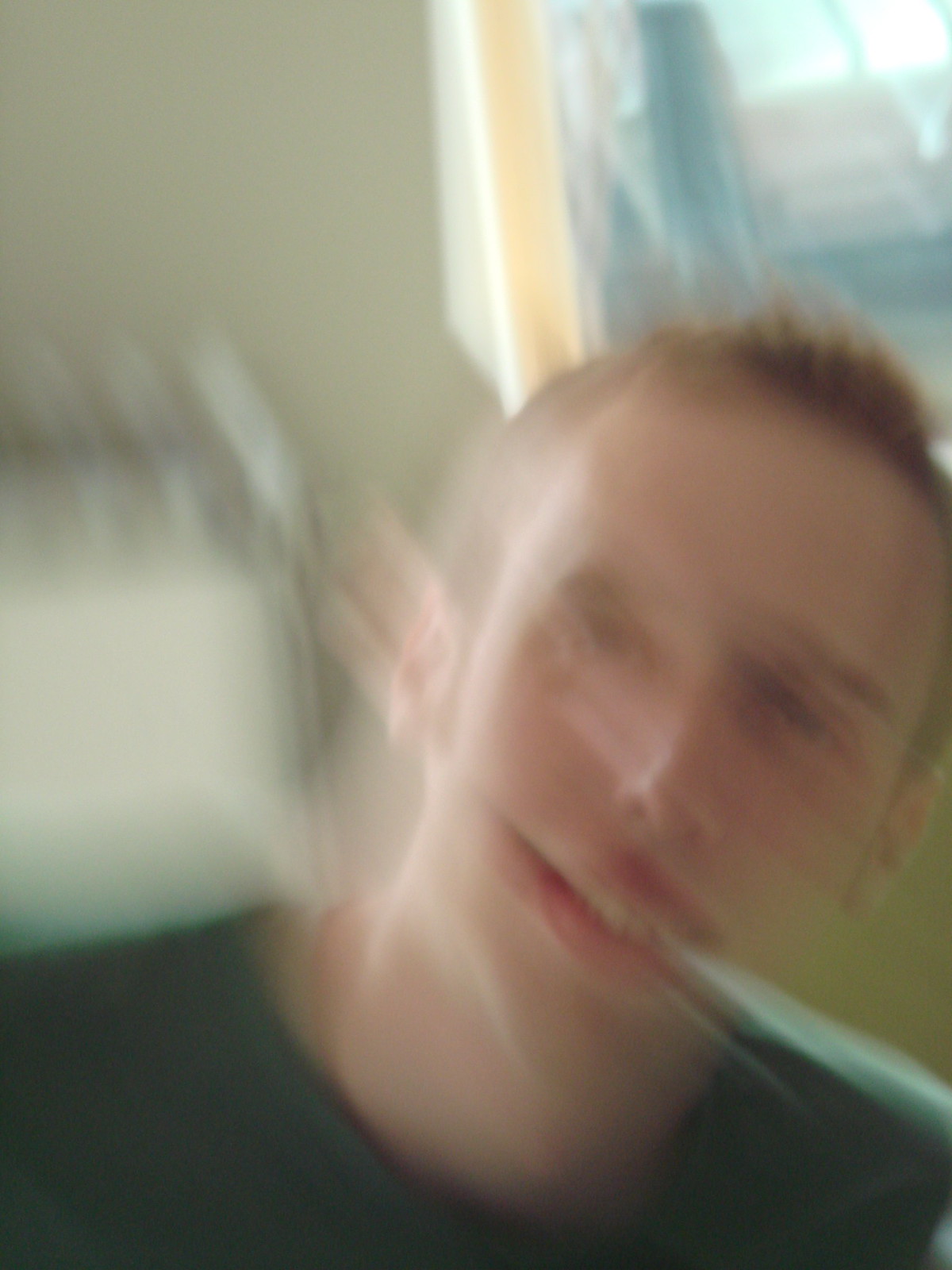The photograph is a very out-of-focus image depicting a young man's face, heavily distorted due to rapid movement. He appears to be in his twenties, with pale skin and short, spiked brown or auburn hair that is cropped on the sides. His face is turned slightly to the right and significantly blurred, with streaks indicating motion. Despite the blurriness, he seems to be smiling, showing a glimpse of his top teeth and thick pink lips. He's wearing what appears to be a green or black t-shirt with possibly another shirt underneath, as indicated by a visible rim around his neck. 

In the background, a white wall can be seen to the left, along with what might be a white door frame. There is also a window or a portrait featuring bright light and potentially a building or tree scene behind him. Additionally, there's a suggestion of a brown, light brown couch off to the side. The overall image gives an impression of a dynamic moment captured in poor focus, with light streaming in from a window and multiple indistinguishable elements in the background.